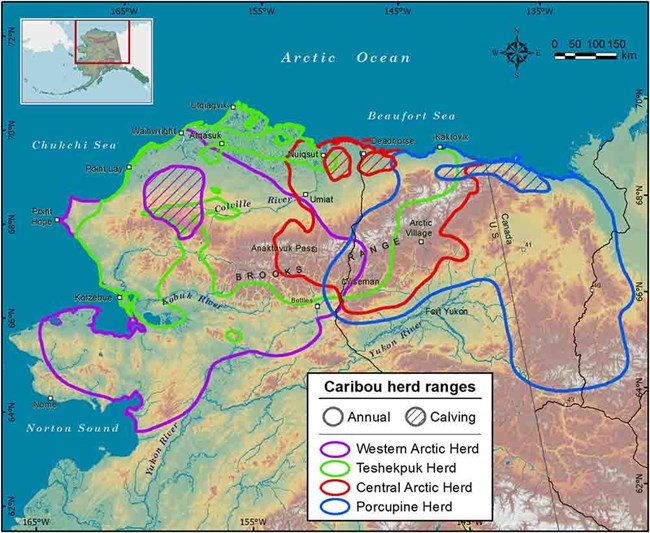This image is a detailed map highlighting the caribou herd ranges across a specified region, likely in Alaska. Prominent at the top of the map, "Arctic Ocean" is inscribed in white text, with the "Beaufort Sea" centrally positioned, and to the left, the "Chukchi Sea" is noted. The map features a compass at the top center, indicating directions (N, W, E, S), accompanied by a scale for kilometers. The map is marked with longitudinal lines at 165°, 155°, 145°, and 135° west. Alongside the landmass, various geographical features like the Brooks Range, Yukon River, and Fort Yukon are illustrated, and the boundary between the USA and Canada is delineated. At the bottom, a key explains the color-coded caribou herd ranges: purple for the Western Arctic Herd, red for the Central Arctic Herd, blue for the Porcupine Herd, and other shades for the Teshekpuk and Annual Calving herds. The map combines hues of blue for the oceans and seas, with browns and greens for land, creating a colorful and informative depiction of caribou movements.